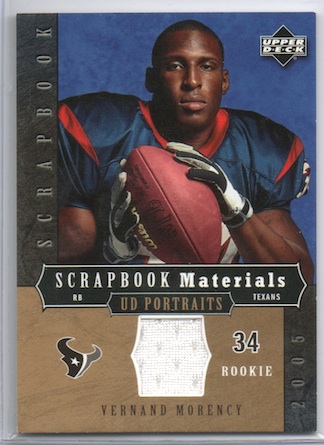The image is a detailed Upper Deck sports card, specifically a rookie football card for Vernon Morency, a player for the Houston Texans. The card features a gray border with a blue background. Vernon Morency is depicted in a dark blue and red jersey, holding a football with both hands, wearing white and black gloves, and staring directly into the camera with an expressionless look. His jersey number, 34, and position as a rookie running back are highlighted. The card has several notable features: the Upper Deck logo in the upper right corner, the word "Scrapbook" written sideways in black on the left side, and "Scrapbook Materials" in white with "UD Portraits" in brown underneath the photo. There is also a brown square featuring a longhorn symbol with a star, indicating a Texas team. Additionally, there is a fragment of his jersey embedded in the card, suggesting it is a patch card from a special release line in 2005 known as "Scrapbook Materials."